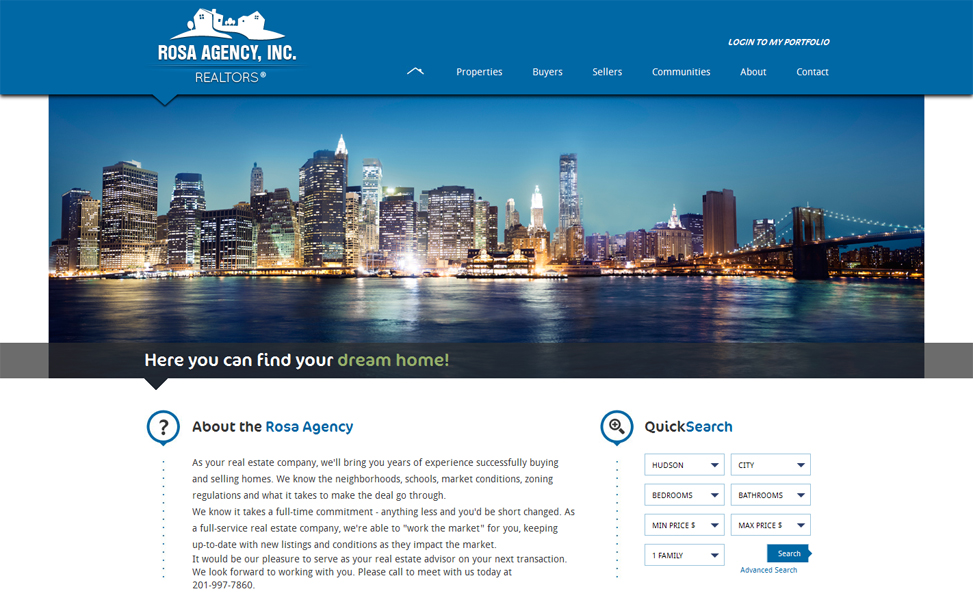Here is a detailed and cleaned-up caption for the image described:

---

The image features a modern and sleek real estate promotional design. The background is primarily blue, providing a calming and professional atmosphere. On the left side, there are generic images of houses and lush green grass, suggesting residential properties. The text "Roja Agency Inc. Realtors and More" is prominently displayed in white, positioned to catch the viewer's attention.

On the right side of the image, a navigation menu lists various options: "Properties," "Buyers," "Sellers," "Communities," "About," and "Contact." Above this menu, the option to "Log into My Portfolio" is available. A stunning city skyline, likely New York City, is featured in the center. This skyline is beautifully lit up, either at dusk or dawn, with a distinguishable bridge on the left and a river running below it, contributing to the urban aesthetic.

At the bottom of the skyline image, a motivational message encourages prospective clients: "You can find your dream home," with the words "dream home" highlighted in a tan color for emphasis.

Below this section, a blue circle with a black question mark signifies more information about Roja Agency, although the detailed text is not clearly readable. To the right, another blue circle contains a black magnifying glass, representing the quick search feature. The phrase "Quick Search" is clearly written next to this icon, with the words "quick" in black and "search" in blue.

Finally, a comprehensive search tool allows users to filter properties by region such as "Hudson City," specify the number of "bedrooms" and "bathrooms," and set "minimum" and "maximum" price ranges. The tool also includes options like "one family." A blue button labeled "Search" in white text invites users to initiate their property search.

---